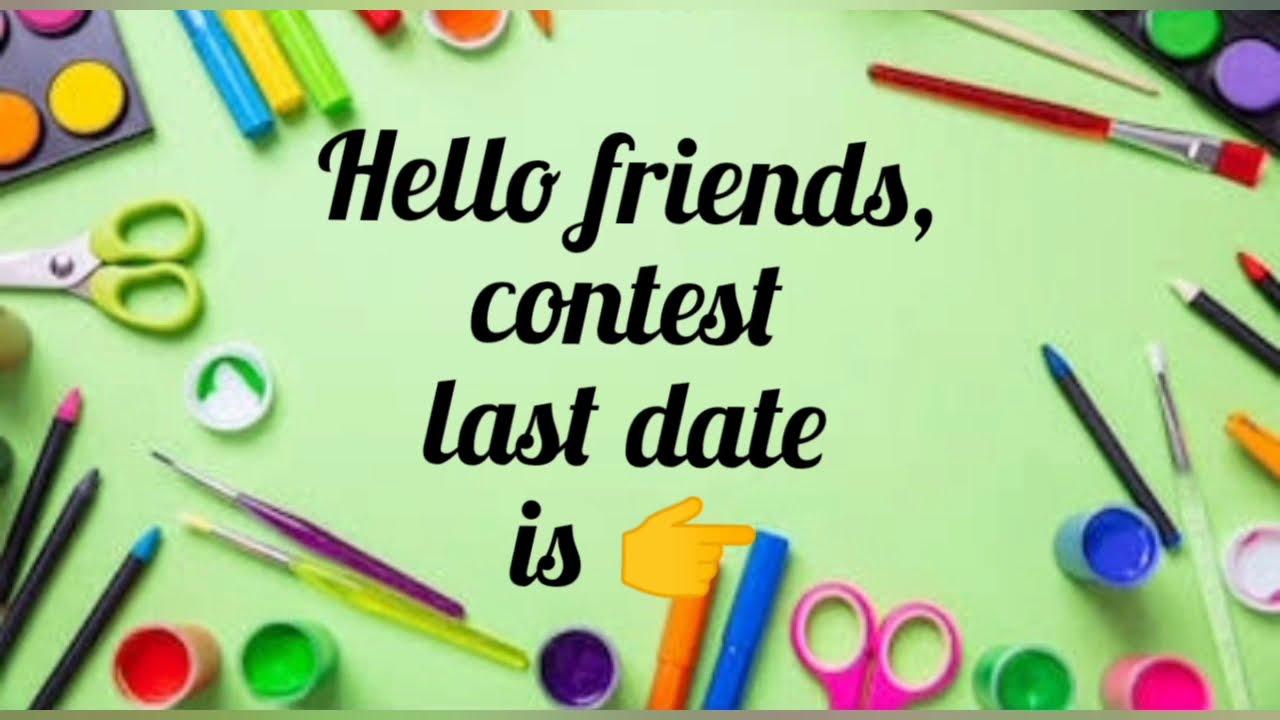The image depicts a vibrant, artsy workspace with a green tabletop scattered with various arts and crafts supplies. In the center, in bold black cursive font, the text reads: "Hello friends, contest last date is," with a yellow hand emoji pointing to the right, indicating where the contest date would be placed.

Surrounding the text are numerous art supplies: a pair of scissors with green handles and another with pink handles, multiple paintbrushes with clear plastic handles—some green, some purple—and several colored pencils with tips in blue, white, and red. Additionally, there are small paint containers filled with colors like red, green, purple, pink, and blue. 

On the upper right side of the image, there's a paint palette containing purple and green paint with a black cover, and on the upper left, another paint container alongside blue, yellow, and green markers. The workspace is lively, indicative of creative activity, drawing attention to the announcement in the middle.